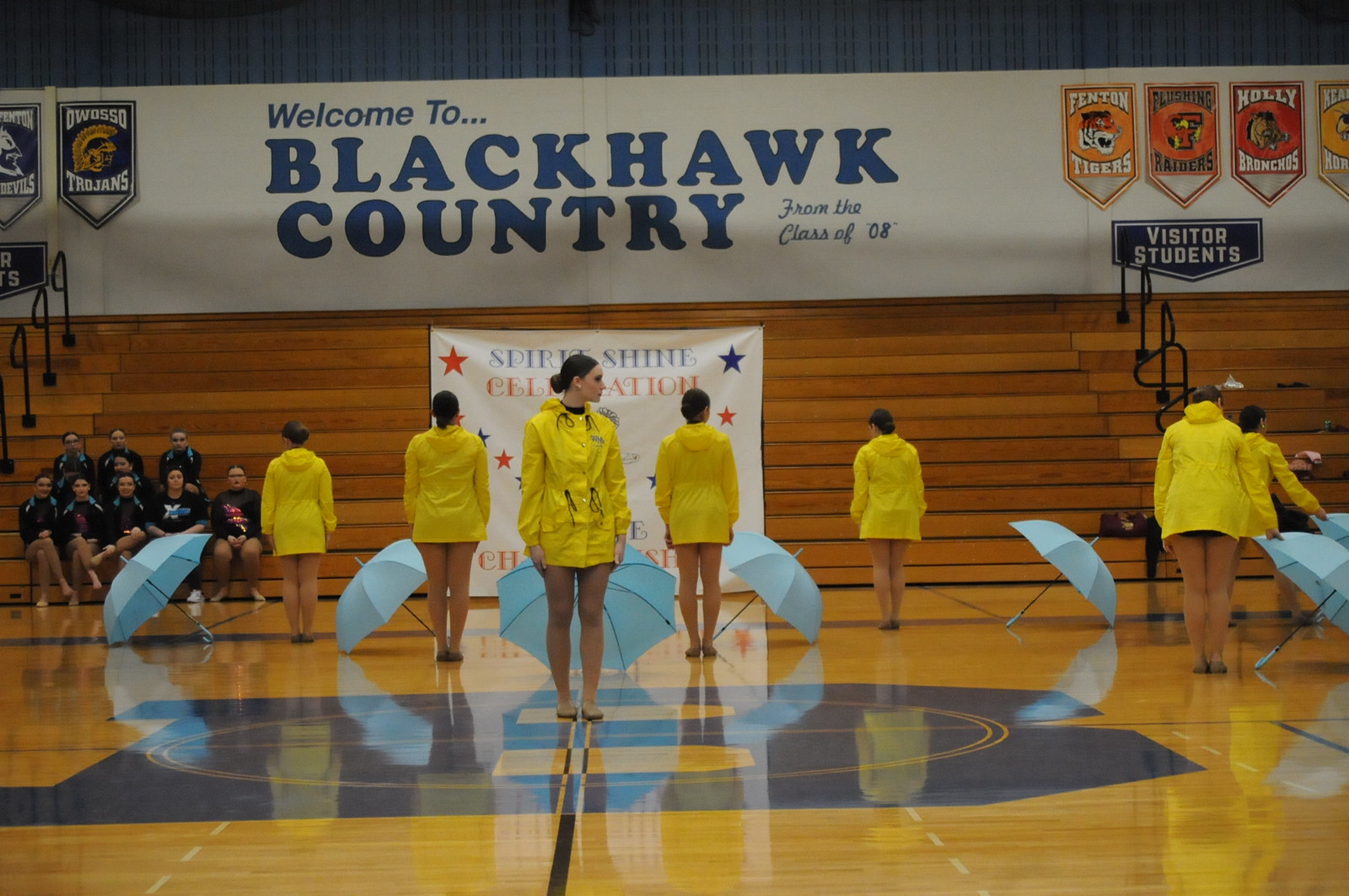The photograph captures a dynamic scene inside a school gymnasium. In the foreground, seven girls, dressed in striking yellow rain jackets that fall to the top of their legs, stand on the gymnasium's shiny, reflective orange-wood floor. The center of the floor features a large, prominent blue "B" logo. Each girl has a blue umbrella, propped open on the ground beside her. The girls appear to be in mid-performance or practice, forming a triangular pattern. Only the middle girl in this formation faces the viewer, though her gaze is directed to the right.

In the background, the gym's wooden bleachers host several spectators, all dressed in black with blue accents, indicating they might be part of another group or team. Above the bleachers, a prominent banner reads "Welcome to Black Hawk Country from the Class of '08," flanked by smaller banners representing various teams, such as the Tigers, Raiders, and Trojans. The wall beneath the banners sports additional placards and possibly cut-off labels for different sections like "visitor" and "students." The overall setting suggests a celebratory or competitive event, with the gym's decor and arrangement reflecting school spirit and community pride.